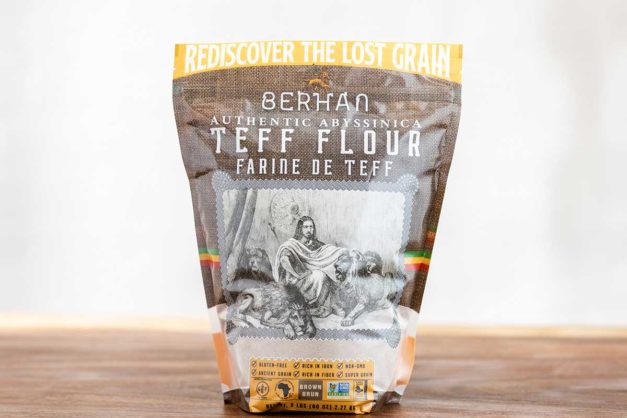In the center of the image, a package of teff flour is prominently displayed on a brown wooden table. The background features a white wall with a gray streak on the right side, giving a bright and clean look. The package has a yellow stripe at the top with the white text "Rediscover the Lost Grain." Below this, the brand name "Berhan" is printed, followed by the words "Authentic Abyssinica Teff Flower." Additionally, the term "Farine de Teff" is noted in French. The lower part of the package features a black and white image depicting a man seated on the ground, flanked by sleeping lions. A yellow label with nutritional information and an icon of the African continent is also visible. The image predominantly uses colors such as green, yellow, red, white, and brown. The teff flour package, the main subject, stands out against the simplistic background, emphasizing its prominence and branding.